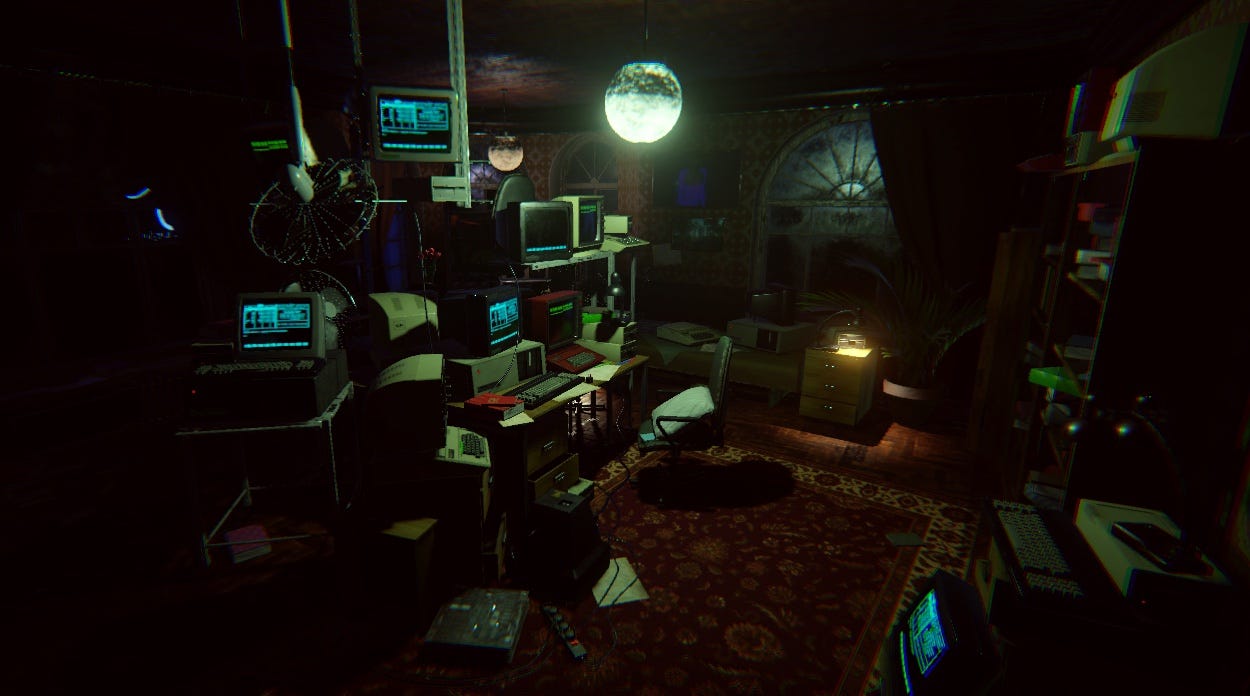The image depicts a dimly lit, dark room filled with old-fashioned computer equipment, predominantly situated on the left side. Several computer monitors and various unidentified devices are arranged under these monitors. Atop the leftmost monitor sits a small desk fan. The floor features a red Persian-style carpet with white-bordered edges, though the intricate pattern is partially obscured by dirt. A brown bookshelf and an additional computer monitor occupy the right side of the room. Towards the back, an arch-shaped window is set above a few file cabinets, one of which supports a lamp. The ambient light in the room comes from a central globe light, casting a pale white hue. The overall clutter of old technology and the dark ambiance make it challenging to discern finer details.